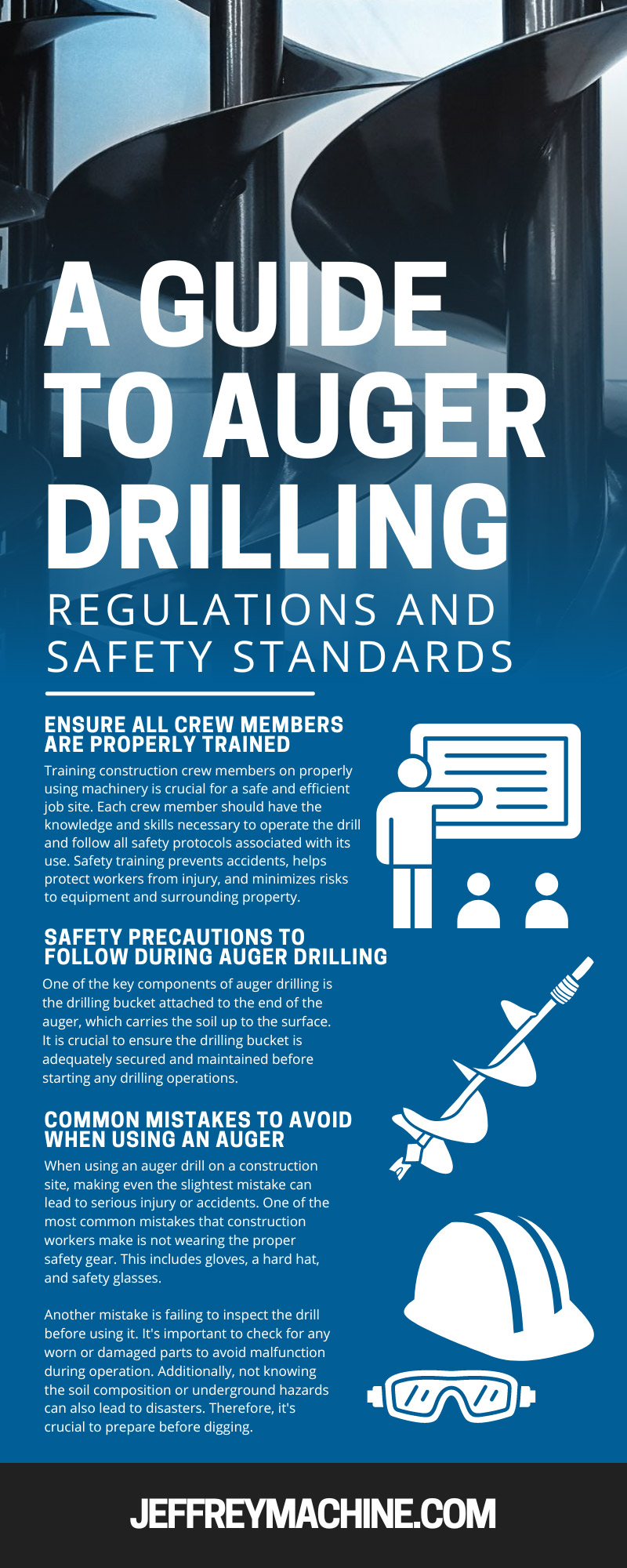This is the front of a pamphlet titled "A Guide to Auger Drilling," produced by jeffreymachine.com, as noted in a black rectangular box at the bottom. The pamphlet features a blue background that fades into a photograph of three auger drills placed side by side at the top. The title is prominently displayed in bold white font, with smaller white text below detailing regulations and safety standards. The pamphlet covers essential topics such as the importance of properly training crew members, safety precautions to follow during auger drilling, and common mistakes to avoid. The right side includes minimalist clipart illustrations of a person presenting to others, a drill, a hard hat, and safety goggles, emphasizing different safety procedures and equipment.